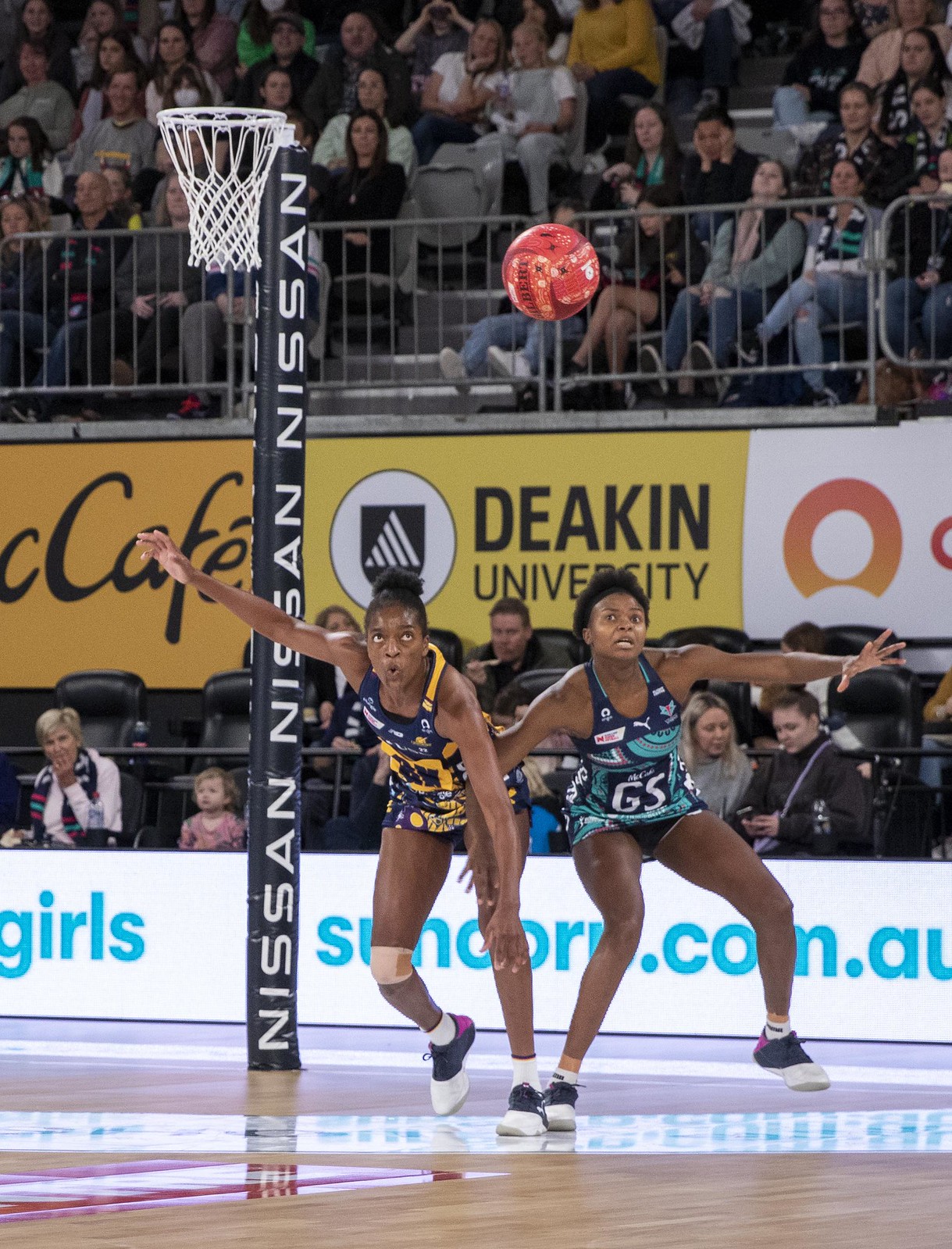This image captures an intense moment of a professional netball game being played indoors at a stadium adorned with various advertisements. Two athletic, dark-skinned women are prominently featured, both fixated on a red and white ball resembling a volleyball in mid-air. The hoop they aim for is distinctive—white with no backboard, mounted on a sleek black pole repeatedly branded with "Nissan." The woman on the left wears a dark blue and gold uniform, while her counterpart on the right sports a light blue and dark blue outfit. Both athletes seem to be in the midst of blocking each other while reaching for the ball. The stadium is bustling with spectators seated on both the lower and upper levels. Notable advertisements adorn the scene, including "Deakin University," "McCafe," and "Girls, Sonora.com AU," enhancing the sporty ambiance of the venue. The court itself is wooden and glossy, reflecting the intense lights, and is likely equipped for high-level netball matches given the professional setup.